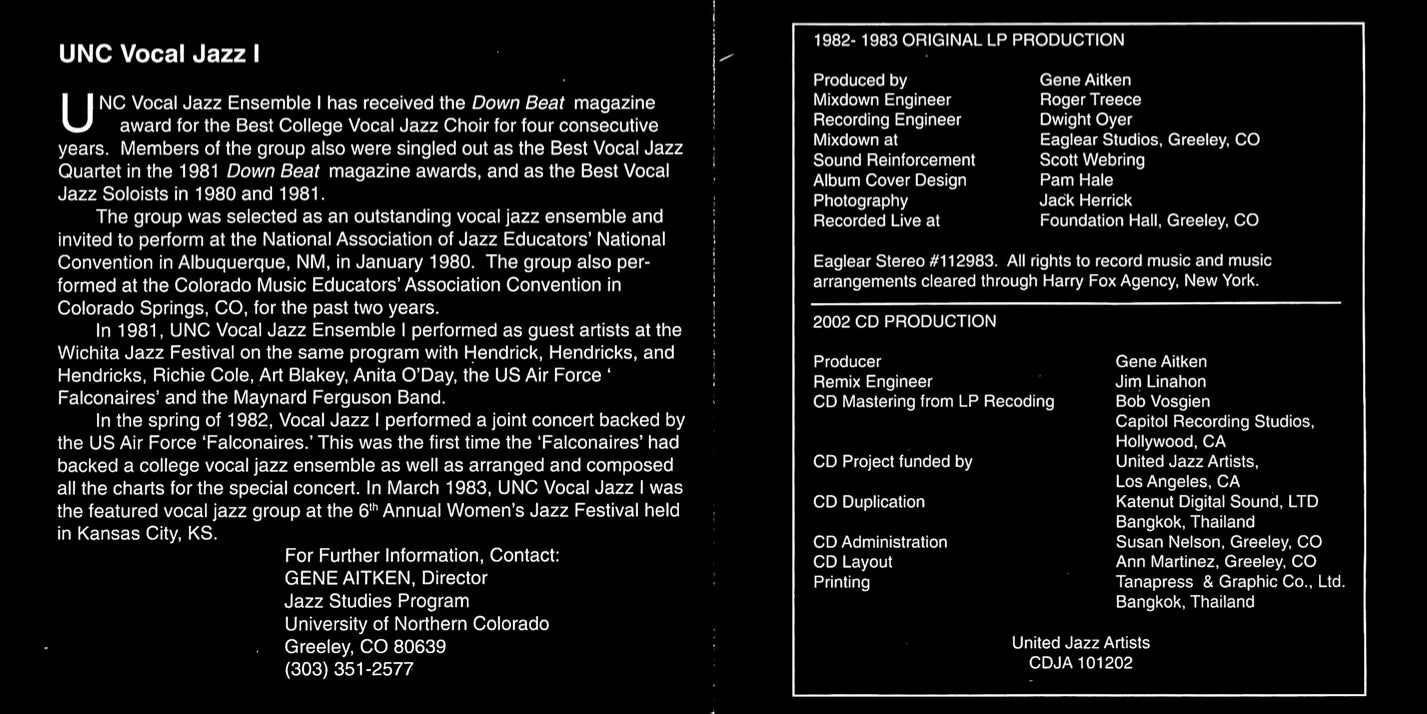The image appears to be the liner notes for a CD reproduction of the original 1982-1983 LP by the UNC Vocal Jazz Ensemble I. The detailed text highlights the ensemble's accolades, including receiving the Downbeat Magazine Award for Best College Vocal Jazz Choir for four consecutive years. The ensemble's members were recognized as the Best Vocal Jazz Quartet in 1981 and the Best Vocal Jazz Soloist in 1980 and 1981. The group was honored as an Outstanding Vocal Jazz Ensemble and invited to perform at significant events, such as the National Association of Jazz Educators National Convention in Albuquerque, New Mexico, in January 1980, and the Colorado Music Educators Association Convention in Colorado Springs, Colorado, for the past two years. In 1981, they performed at the Wichita Jazz Festival alongside notable artists like Richie Cole, Art Blakey, Anita O'Day, the US Air Force Falconaires, and the Maynard Ferguson Band. In the spring of 1982, they held a joint concert with the US Air Force Falconaires. The right section of the notes details the CD's production, listing the original LP production credits from 1982-83 and indicating that it was published by United Jazz Artists. Further information is available by contacting Jean Atikin, Director of the Jazz Studies Program at the University of Northern Colorado.